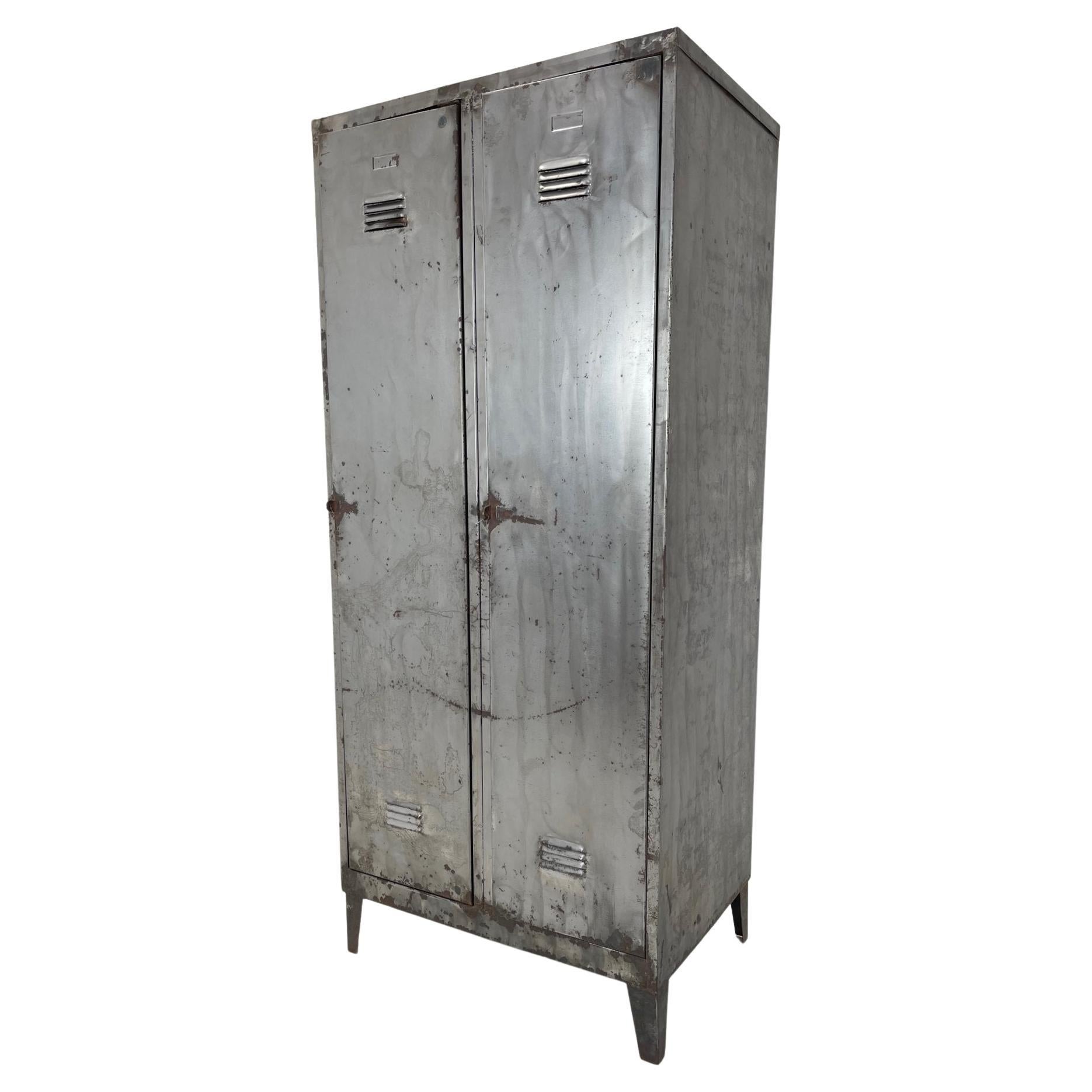The photograph showcases a pair of vintage, stainless steel lockers likely dating from the 1920s to the 1940s. These tall, gray metal lockers stand on four feet and feature double ventilation slots, with vents positioned at both the top and bottom of each door. The storage unit is notably scuffed and dented, indicative of its age and extensive use, though remarkably free of rust. Its surfaces are unpainted and darkened, with a few patches of dirt and wear more pronounced at the bottom. The locker doors lack handles, instead having simple, possibly janky mechanisms, though it’s unclear if locking functions are intact. Set against a plain white background, the image is slightly distorted due to a wide-angle lens.